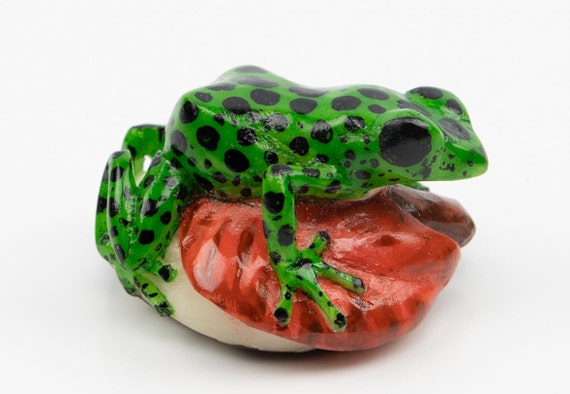The image captures an exquisitely detailed small sculpture, possibly handmade, depicting a vibrant green frog with black dots adorning its body. The frog, characterized by its large, expressive black eyes, is perched atop a striking red object. This object appears to be either a stone, leaf, mushroom, or shell; it has a white base transitioning to an orange-red top with dark red spots. The scene is set against a stark white background, enhancing the vibrancy of the sculpture. The frog is oriented in a profile shot, seemingly poised to leap, staring intently towards the right. The entire piece is rendered in a highly detailed, colorful fashion, suggesting it could be made of either glass, clay, or ceramic, and is likely a small, intricate art piece measuring around six by five inches. Shadows cast by the sculpture add a subtle depth to the otherwise plain backdrop.